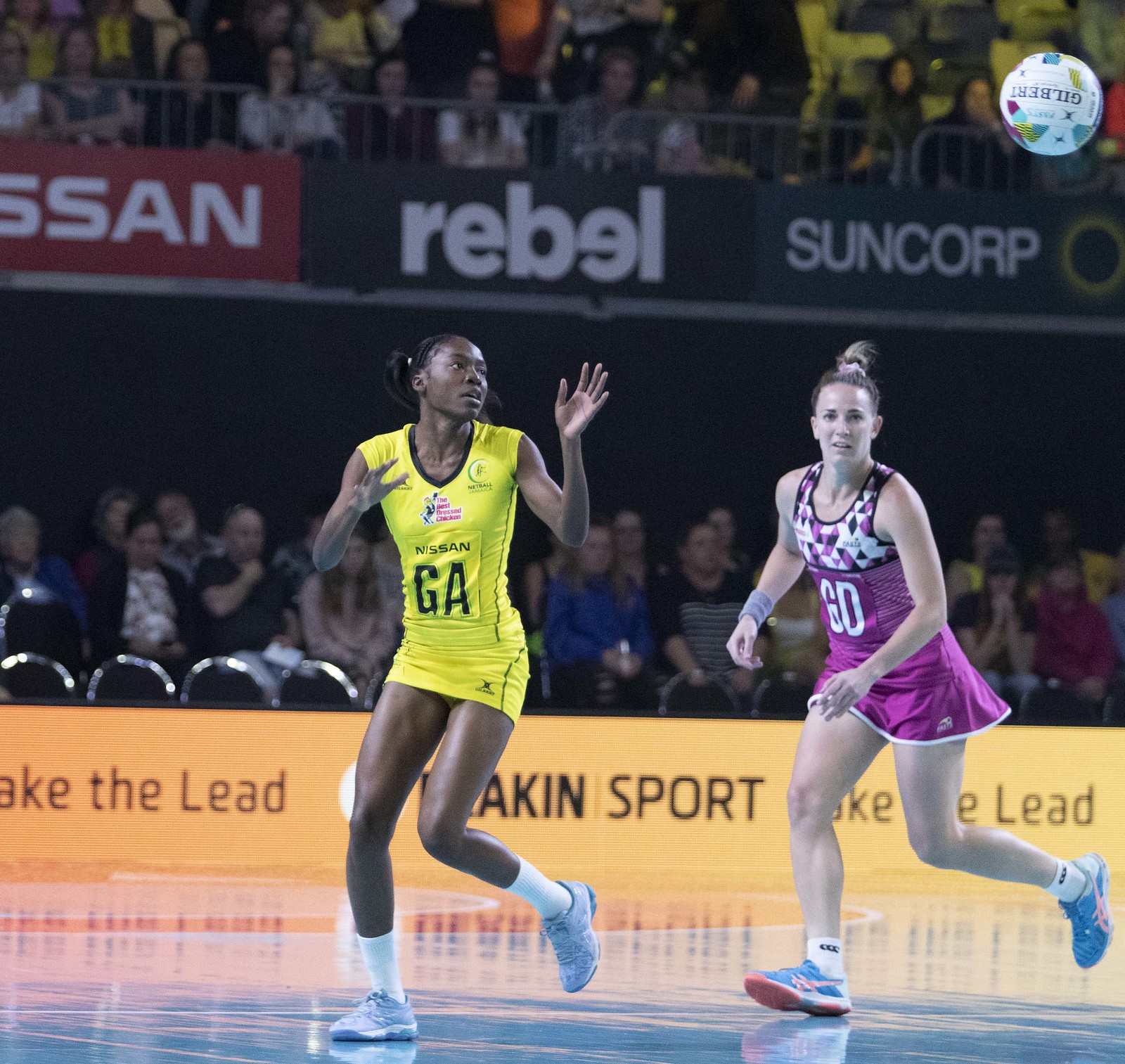The image depicts an intense volleyball game, captured inside an auditorium. The scene is dominated by two female athletes on the court, both caught in mid-action. The player on the left is an African American woman, dressed in a striking yellow athletic outfit that closely resembles a mini-skirt. Her uniform prominently displays the sponsorship logo "Nissan" alongside the large black letters "GA". She is focused and looking upwards towards a volleyball that's suspended in the air, positioned in the upper right-hand corner of the frame. 

Adjacent to her is a white woman clad in a pink athletic dress with white accents, which also functions as a sports uniform. This outfit bears the letters "GD" and she sports multi-colored sneakers in blue and orange. Surrounding the court, spectators fill the stands, which are arranged in two levels, sitting on brown chairs and eagerly watching the match unfold. In the backdrop, various advertisements are visible, including fragmented slogans like "Take the lead" and the brands "Nissan", "Rebel", and "Suncor".

Overall, the vibrant athletic apparel of the players, along with the energetic atmosphere created by the audience and visible branding, underscores the competitive spirit and dynamic action of the volleyball game.